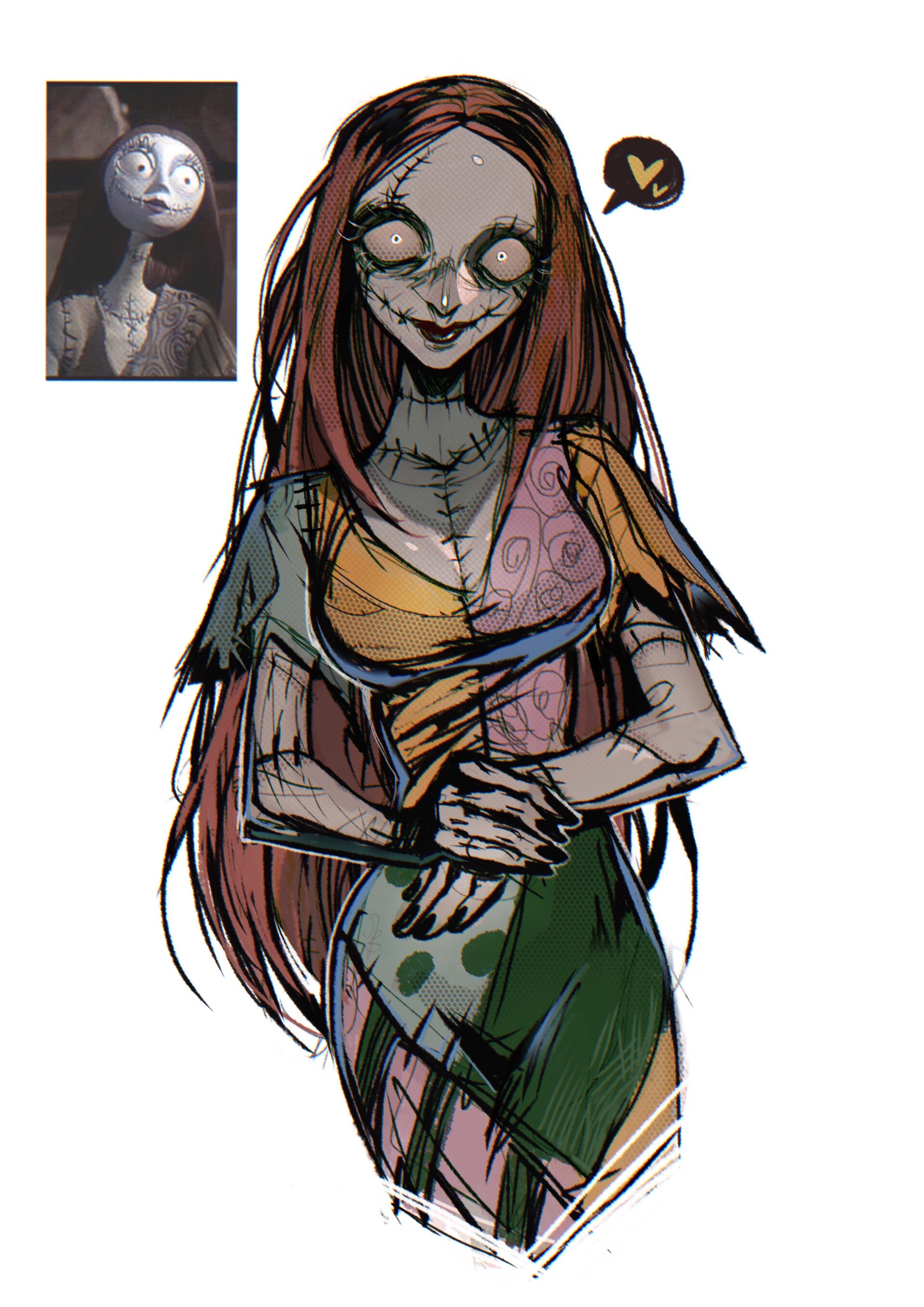The image is a detailed vertical illustration of a character believed to be Sally from Tim Burton's 1993 stop-motion film, "The Nightmare Before Christmas." In the upper left corner, there is a small depiction of Sally as she appears in the original movie, serving as a reference. The main focus of the image is a larger, hand-drawn or digitally created interpretation of the character, emphasizing more stylized and possibly sexualized features. Sally has long, auburn-reddish hair, and her skin is a pale, grayish-brown color with visible stitching marks across her forehead, mouth, neck, chest, and arms, highlighting her patchwork nature. She’s wearing a tattered dress with a plunging neckline, featuring a mosaic of colors such as light gray-blue, green, pink, muted orange, and decorative patterns including flowers, swirls, and polka dots. Her black-painted nails are visible as her hands rest on her abdomen. She has tiny pupils in her large eyes, which are directed at the viewer, and a small smile or smirk on her face. Additionally, there is a speech bubble to the right with two hearts inside, adding a whimsical touch to the illustration.